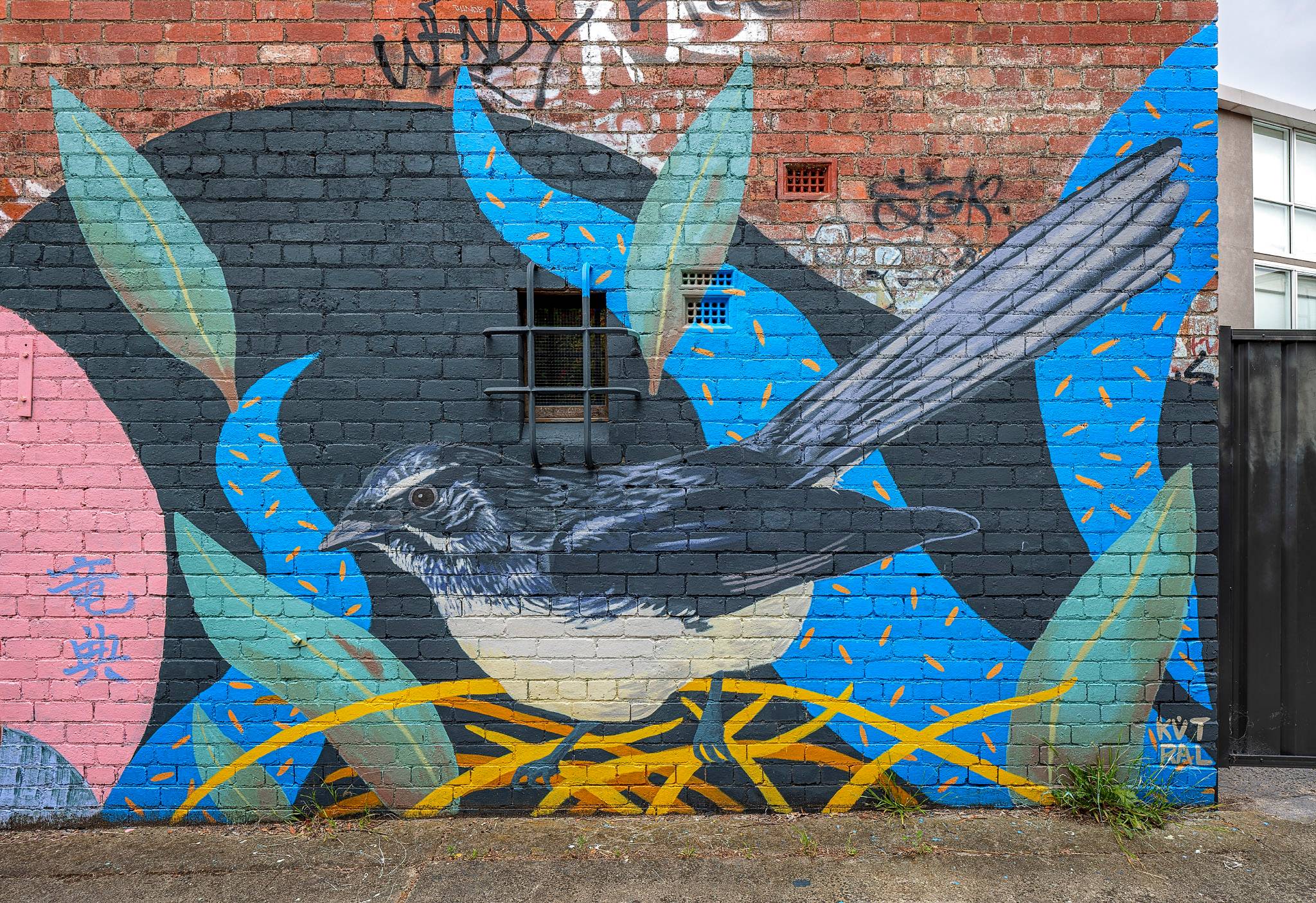The mural is painted on the worn, brown-red brick wall of an old building. The focal point is a large bird, approximately the length of about three people. The bird's upper body, wings, and tail are primarily black, with some bluish hues, while its legs and feet are dark blue. It has a distinctive white stripe over its eye, which blends into a white chest and underbelly. The bird stands on golden, vine-like branches. The background features wavy, turquoise-blue and green leaves with yellow specks, giving the sense of foliage. One leaf appears to be falling behind the bird. The mural also includes blue plants on a black backdrop, along with blue Chinese writing on the left side and a pink painting with blue Chinese characters in the far left corner towards the bottom. There are also some pink shadings and black cursive signatures from the artist.